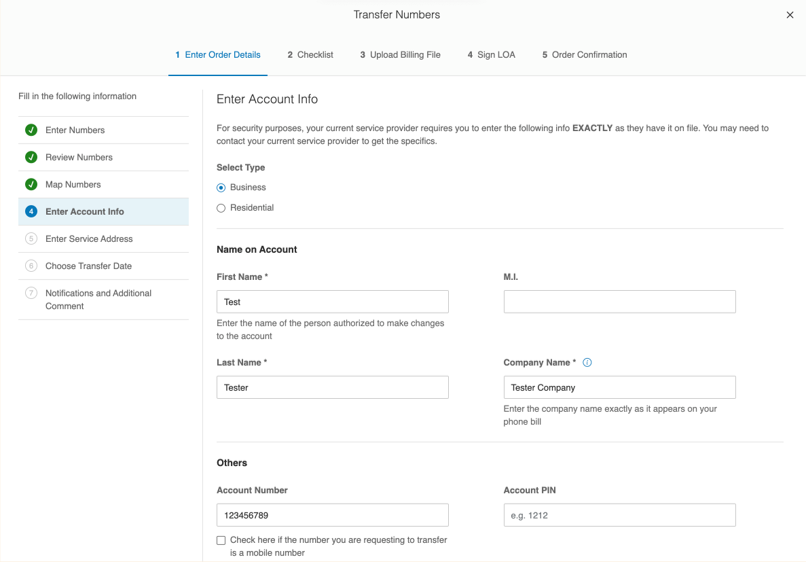In the image, there is a web page featuring a user interface for transferring numbers. The top of the page has a light grayish-blue bar with black text centered within it, reading "Transfer Numbers" with both 'T' and 'N' capitalized. Below this bar, there are five steps listed: 

1. Enter Order Details
2. Checklist
3. Upload Billing File
4. Sign LOA
5. Order Confirmation

Each step is outlined, but only Step 1, "Enter Order Details," is currently selected, indicated by a blue bar underneath it.

On the left side of the page, a progress tracker shows the levels of completion, each with a corresponding green circle and white checkmark except for the current step, which is highlighted with a blue circle and white number:

- "Enter Numbers" - completed
- "Review Numbers" - completed
- "Map Numbers" - completed
- "Enter Account Info" - in progress, marked in blue
- "Enter Service Address" - pending
- "Choose Transfer Date" - pending
- "Notifications and Additional Comments" - pending

In the main section of the page, the current task is "Enter Account Info," which requires the user to enter precise details as held by their current service provider. Bold instructions emphasize accuracy, noting that specifics must match the provider's records exactly.

Users are prompted to "Select Type," with choices between "Business" and "Residential." The "Business" option has been selected, and a blue circle marks this choice. Below is a gray line separating it from the next section.

The form requests several details:

- **First Name** (with an asterisk indicating a required field) - "TEST" is entered.
- **Middle Initial** - not entered.
- **Last Name** (required) - "TESTER" is entered.
- **Company Name** (required) - "TESTER COMPANY" is entered, with an information icon next to it, specifying to enter the name exactly as it appears on the phone bill.

Another gray line follows, leading to the "Others" section, marked with a capital 'O'. Here, it asks for:
- **Account Number** - "123456789" is entered.
- **Account PIN** - "1212" is entered.

There is a checkbox option saying, "Check here if the number you are requesting to transfer is a mobile number," but this has been left unmarked.

Finally, in the upper-right corner of the page, there is an 'X' icon to close out the screen.